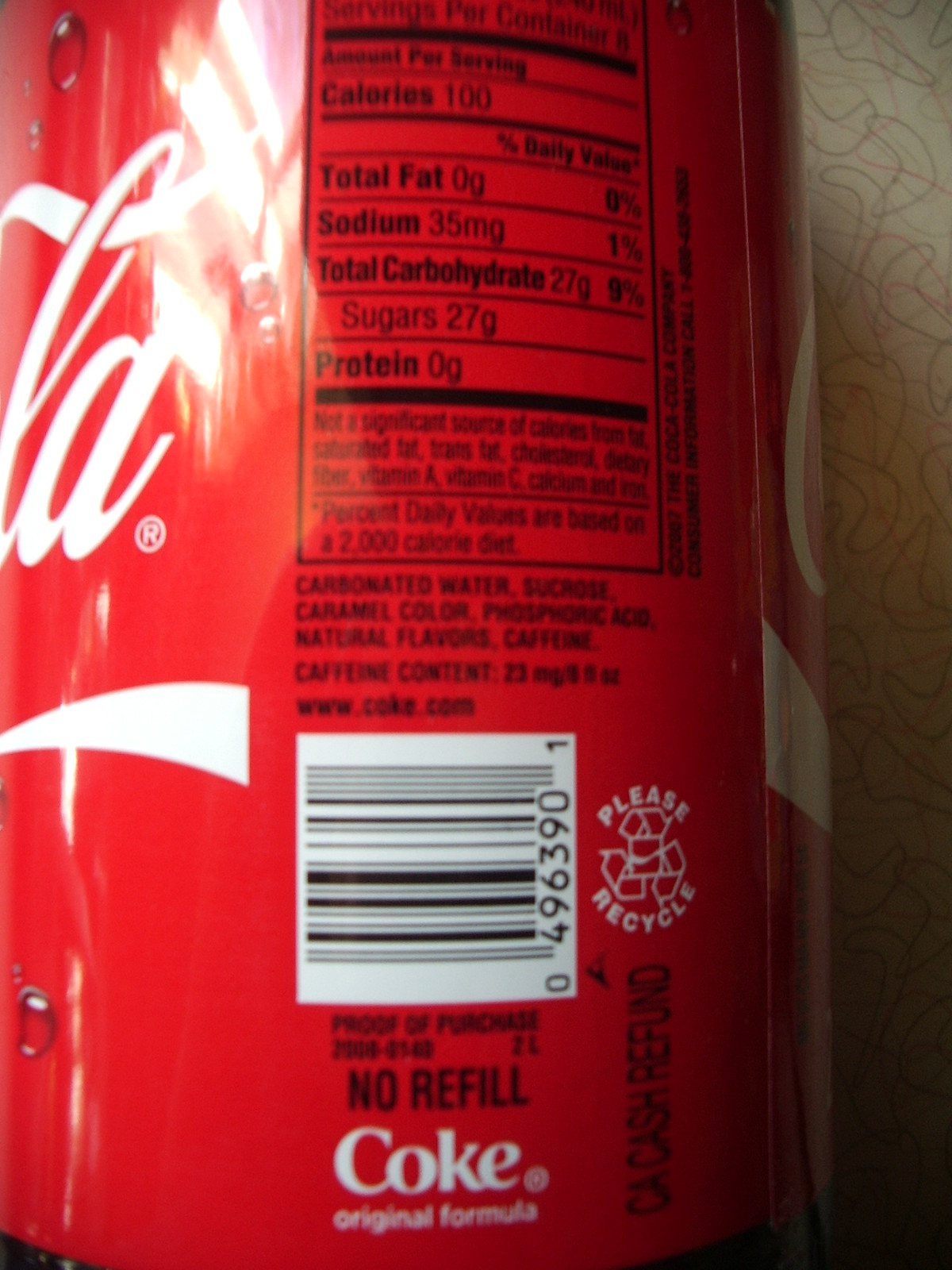The image captures a detailed view of a Coca-Cola can from the Coca-Cola Company. The perspective focuses on the side panel of the can. To the left, only the letters 'L' and 'A' from the iconic Coca-Cola script are visible with a line beneath them, while the right side shows the beginning of the 'C'. The main emphasis is on the nutritional information section. This can contains 100 calories per serving, with no fat, 35 milligrams of sodium, 27 grams of carbohydrates, 27 grams of sugars, and no protein. 

Further information indicates that the beverage is not a significant source of other nutrients. The listed ingredients include carbonated water, sucrose, caramel color, phosphoric acid, natural flavors, and caffeine, with a caffeine content ranging from 20 to 23 milligrams per 8 ounces. The Coca-Cola website is provided, www.coke.com, located above the barcode, which is accompanied by the universal recycling symbol with the words "please recycle" inscribed around it. Additionally, there is a mention of a C.A. cash refund, indicating monetary returns for recycling in certain areas.

Below the barcode are the terms "proof of purchase" followed by a sequence of numbers, the phrase "no refill," and the word "Coke" with a registered trademark symbol. The can also specifies "original formula" in very small letters, affirming its classic recipe.